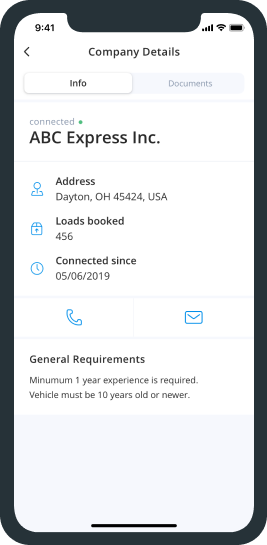Here’s a detailed caption for the image described:

---

The screenshot is taken on a cell phone displaying a page titled "Company Details." At the top, there are two tabs: "Info" in black text on a white bar, and "Documents" in blue text on a light blue or grayish bar. Below the tabs, in tiny gray text accompanied by a small green dot, it says "Connected." Beneath this, in bold black text, the company name "ABC Express, Inc." is listed, followed by the address: "Dayton, Ohio, 45424, USA." The next line provides the statistic "Loads Booked: 456," and another line indicates "Connected Since: 05-06-2019." 

Further down, there are two clickable blue icons, one resembling a telephone and the other an envelope. Below these icons, the section "General Requirements" is outlined, stating that a "Minimum one-year experience is required" and "Vehicle must be 10 years old or newer." 

Additionally, standard mobile interface details are visible at the top of the screen. The time is shown in the upper left corner as "9:41," while the upper right corner displays four signal bars, a Wi-Fi symbol, and a battery icon, all in black.